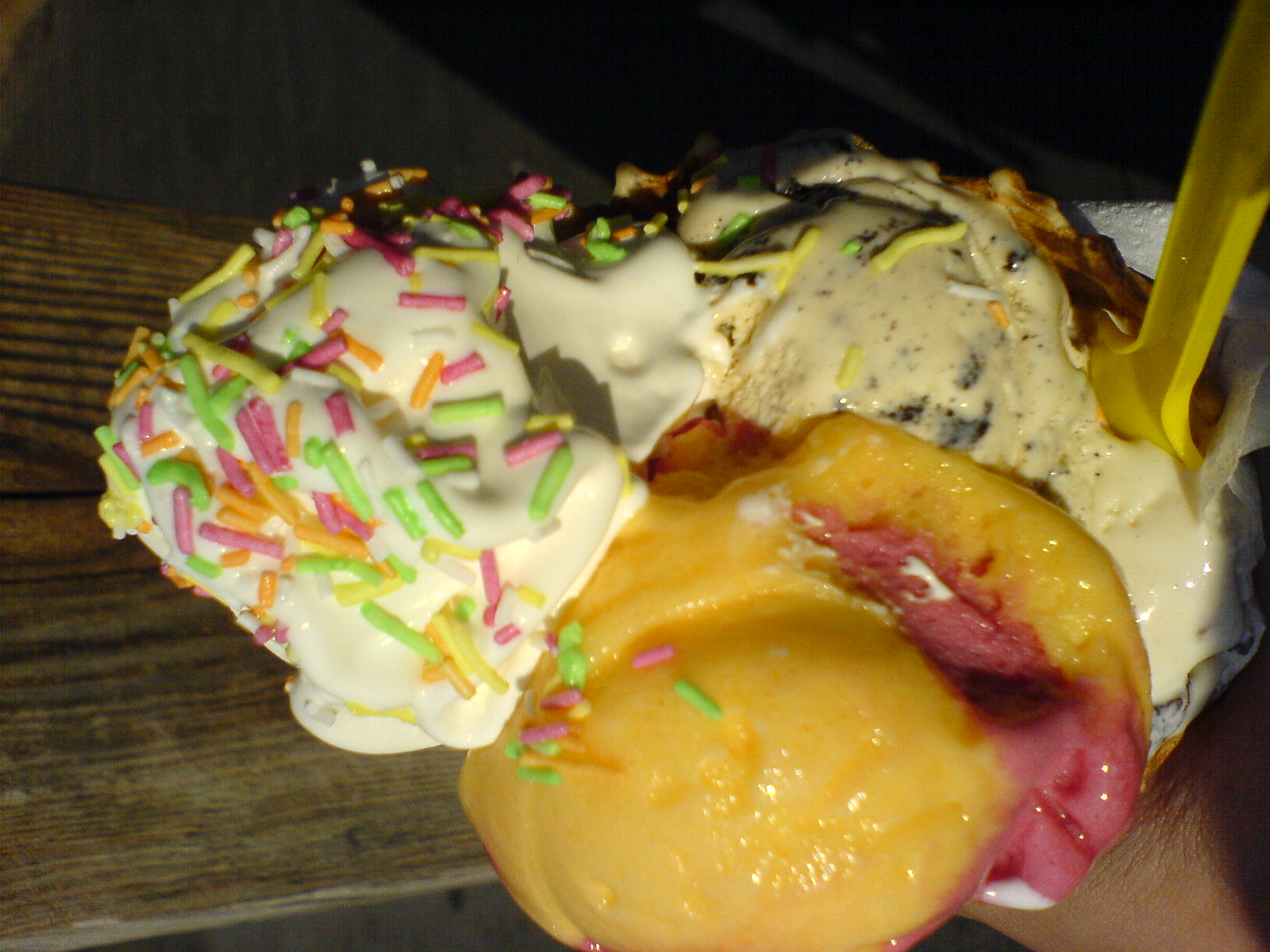This detailed close-up photograph captures a mouthwatering dessert ensemble of three distinct scoops of ice cream nestled in a waffle cone. The first scoop is a classic vanilla adorned with a vibrant medley of lime green, yellow, and pink sprinkles. The second scoop, embodying a sherbet-like consistency, is a blend of yellow and pinkish-raspberry hues, suggesting a delightful combination flavor. The third scoop is cookies and cream, characterized by its off-white base punctuated with substantial chocolate cookie chunks. Completing the scene is a bright yellow plastic spoon poised in the ice cream, indicating a moment ready for indulgence. The hand holding the cone is wrapped in a white napkin, hovering over a rustic outdoor picnic table, adding a touch of everyday charm to this delicious snapshot.